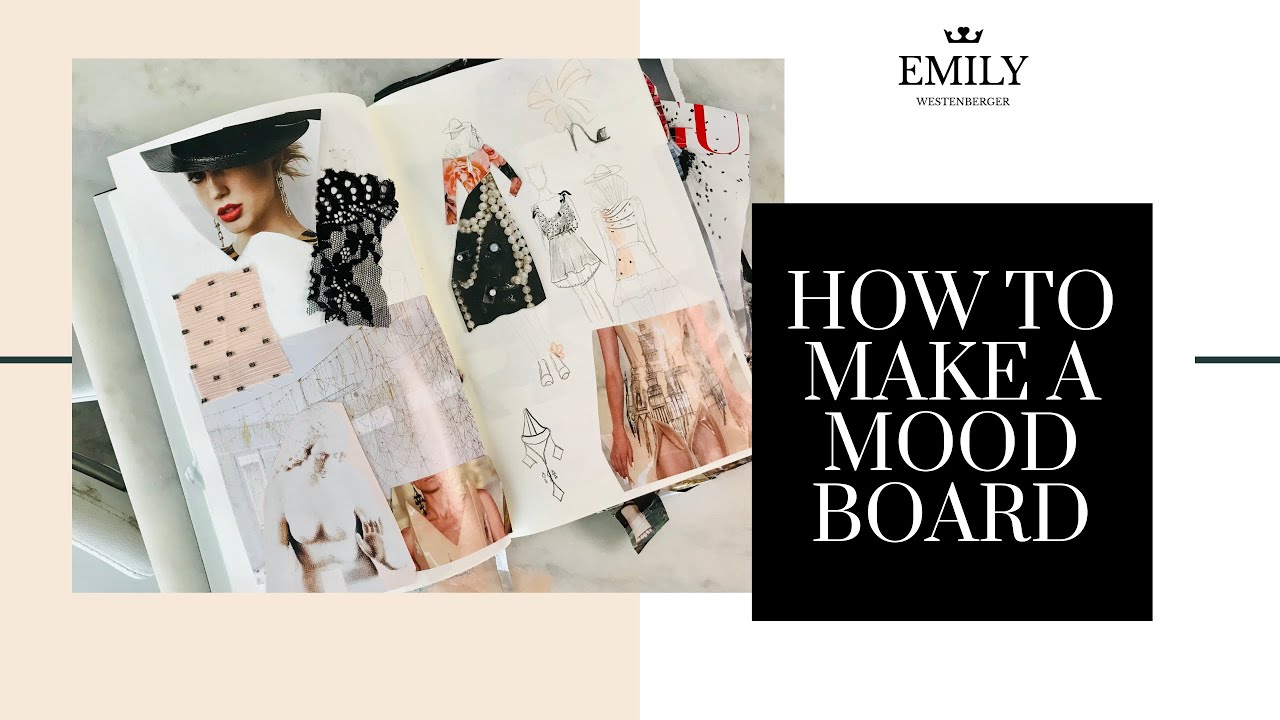The image depicts a digital poster with a white background. On the right side, there is a large black square featuring white text that reads "How to Make a Mood Board." Just above this black square, on the white background, is a smaller print that includes a crown icon, followed by the name "Emily Westenberger." On the left side of the poster, there is a large pink square overlaying the white background. Centered on this pink square is a picture of an open book or scrapbook resting on a flat surface. The book's pages contain a collage of various elements: a photograph of a woman in a black hat with a veil, snippets of black lace and pink dotted fabric, illustrations of shoes and dresses, and a drawing of a woman in a black skirt and red top. Additionally, there are pictures of a naked bust and various other garment designs and textures. The overall impression is that of a mood board or design book filled with a mix of photographs, fabric samples, and sketches.